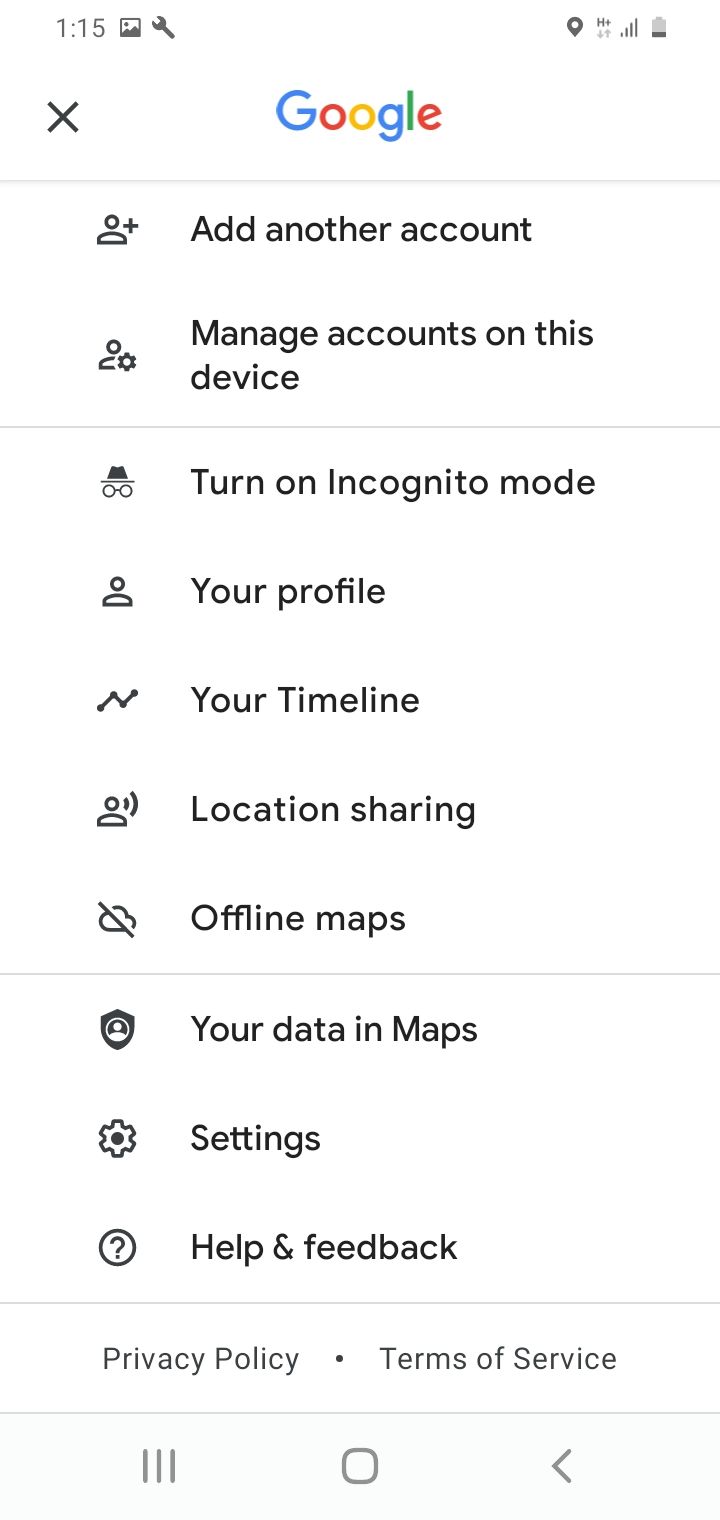The image is a mobile screenshot displaying Google's account settings panel. The panel has a white background and features the Google logo prominently at the top center, with an "X" button for closing the panel located on the far left. Beneath the Google logo is a vertical list of settings options. Each option has a corresponding icon on the left side, with the title of the setting positioned to the right of the icon.

The first entry at the top of the list features a profile icon with a plus sign to its right, labeled "Add another account." The next option is "Manage accounts on this device," followed by "Turn on Incognito mode," "Your profile," "Your timeline," "Location sharing," "Offline maps," "Your data in Maps," "Settings," and finally "Help & feedback."

At the very bottom of the screen, on the left side in small gray font, it says "Privacy Policy," while on the right side it says "Terms of Service," also in small gray font. Below these text entries, the screenshot reveals the phone's navigation options, including a menu icon on the far left, a square icon in the center to minimize the page and return to the home page, and an arrow button pointing to the side on the far right for additional navigation functions.